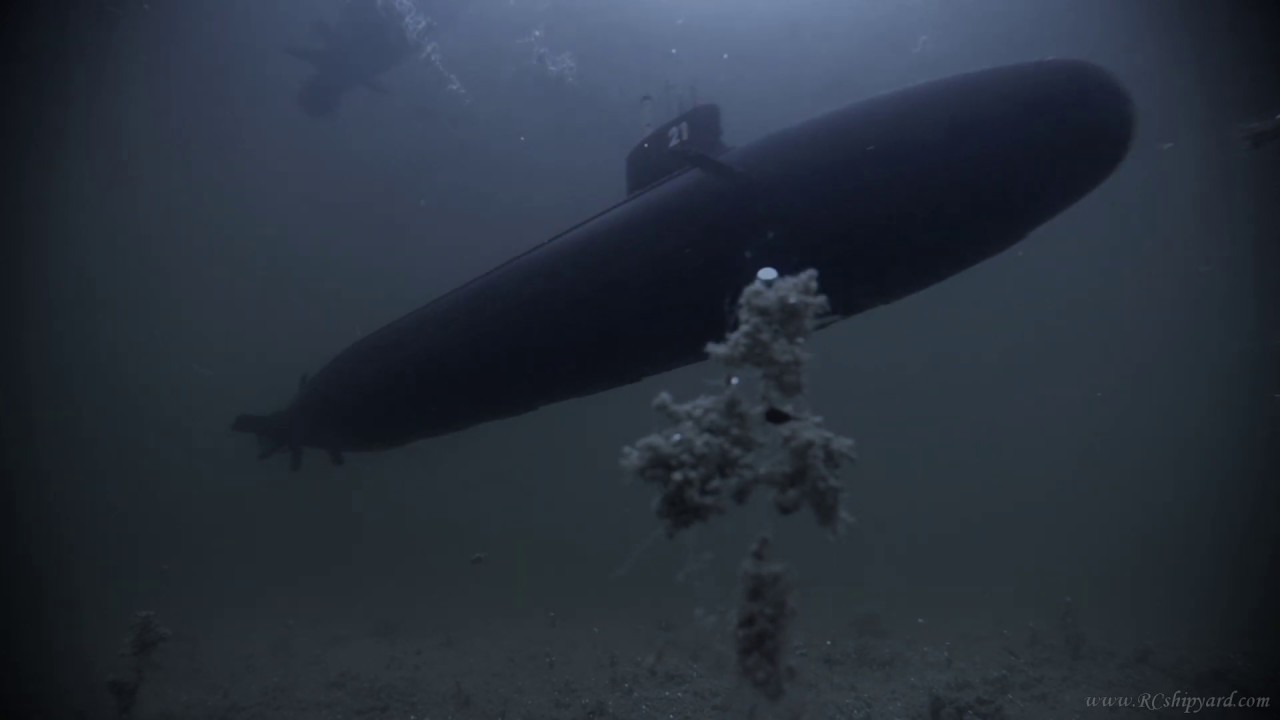The photograph captures a large, dark submarine, identifiable by the number 21 printed near the top, immersed in murky, muted waters. The overall scene is somewhat blurry and dim, with a color palette dominated by dark blue, light blue, black, and grayish tones. Above the submarine, a few air bubbles ascend through the water, while a vague dark shape, possibly a diver's reflection, lingers at the top left. Below, there's a distortion area featuring shapes that could be underwater foliage, thick bubbles, or movement in the water. Additionally, elements resembling underwater vegetation or algae are seen floating near the submarine. In the bottom right-hand corner of the image, the website www.rcshipyard.com is visible.